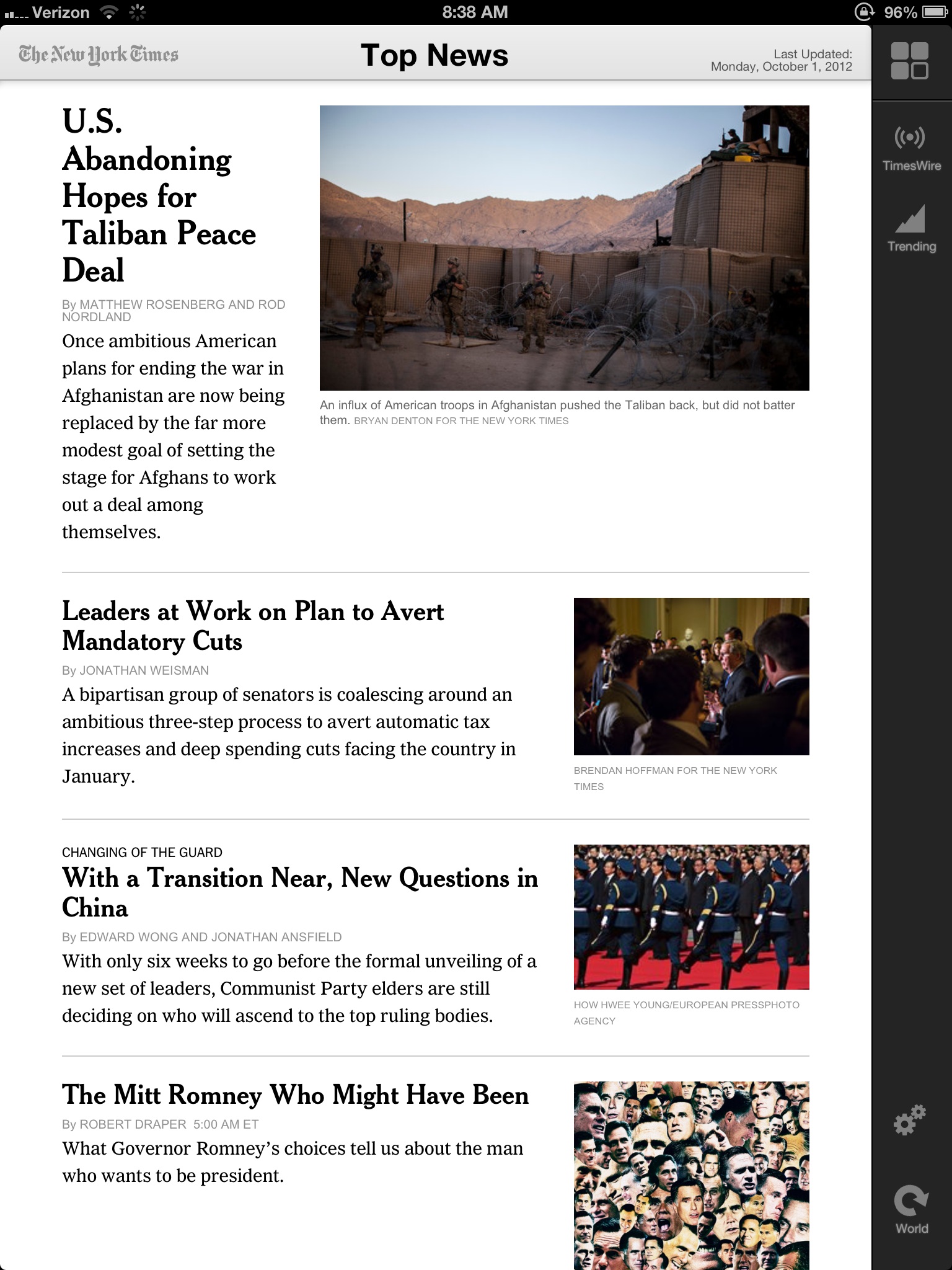This image, sourced from the New York Times online and viewed on a cell phone, features a series of insightful articles. At the top, "U.S. Abandoning Hopes for Taliban Peace" headlines an article discussing the geopolitical challenges and includes an evocative picture of military personnel guarding an area near rugged mountains. Below, another headline, "Leaders at Work on Plan to Avert Mandatory Cuts," signals efforts to navigate fiscal constraints. The next article, "With a Transition Year, New Questions in China," examines the uncertainties surrounding China’s new leadership phase. Finally, "The Mitt Romney Who Might Have Been" reflects on Romney’s political choices with a headline that reads, "What Governor Romney's Choices Tell Us About the Man Who Wants to be President." Each article comes with a respective thumbnail image, enriching the visual and contextual experience for the reader.